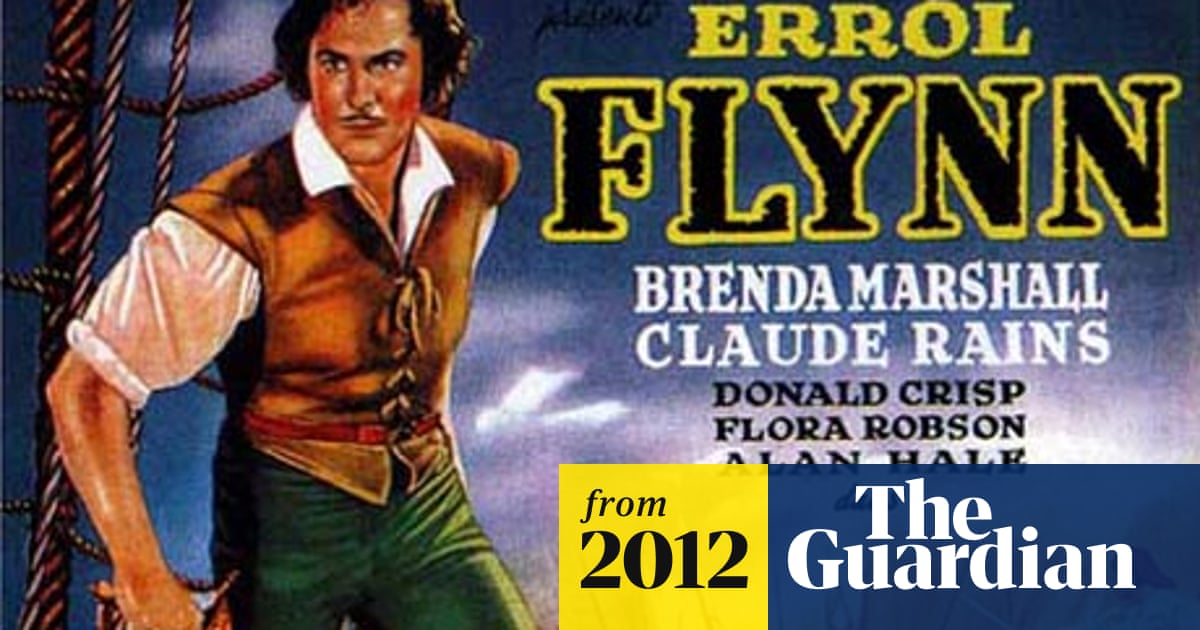In this vivid color poster, prominently featured in yellow text is the name Errol Flynn, outlined in yellow with a dark fill. Directly beneath, in white letters, are the names Brenda Marshall, Claude Rains, Donald Crisp, Flora Robson, and Alan Hale. The poster, which appears to be an advertisement for a movie, segments the names neatly across the top and bottom sections. Errol Flynn is illustrated on the left side, clothed in a red or brownish-orange laced-up vest over a white shirt, with green pants. His sleeves are rolled up above his elbows, exposing a white shirt collar hugging the vest. Flynn’s character appears rugged, with long dark hair, a delicate mustache, bushy eyebrows, and reddened cheeks. He gazes off to the left, grasping some braided ropes, indicative of a ship setting, possibly suggesting a pirate-themed narrative. The background blends hues of blue with subtle white. Toward the poster’s bottom right corner, within a small blue box, are the white text “The Guardian,” and beside it, in black text within a yellow box, the year 2012, hinting at the publication source.